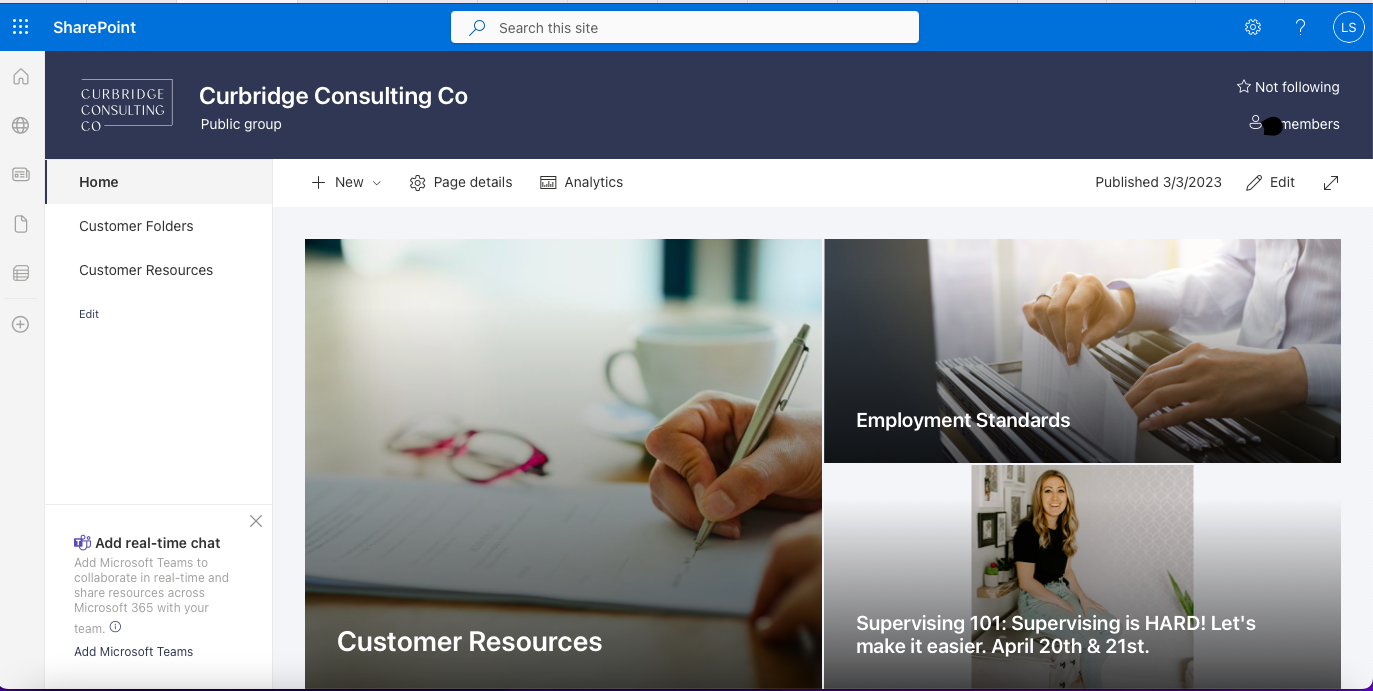**Caption: SharePoint Interface for Kerbridge Consulting Company Public Group**

The SharePoint interface for the Kerbridge Consulting Company Public Group is prominently displayed. At the top, a blue navigation bar bears the title "SharePoint." On the far left of this bar is a grid icon, which, when clicked, reveals a grid image. Centrally located, a search bar invites users to "search this site." To the right, there are icons for settings, a help question mark, and the user's initials "LS" encased in a circle.

A vertical sidebar on the left offers quick navigation options including Home, Web, Documents, Word, and an additional functionality accessible via a plus sign.

Beneath the primary blue bar is a darker blue-gray bar stating "Kerbridge Consulting Company Public Group," which indicates that the user is "Not Following" this group. The bar also shows the number of members, although the exact figure is obscured. 

Below this, navigation options such as Home, New, Page Details, Analytics, and the publish date—March 3, 2023—are listed. There are also options to edit the page or view it in full screen.

The main content area features images of people engaged in various activities like filing documents and writing on notepads, accompanied by a prominent photo titled "Supervising 101."